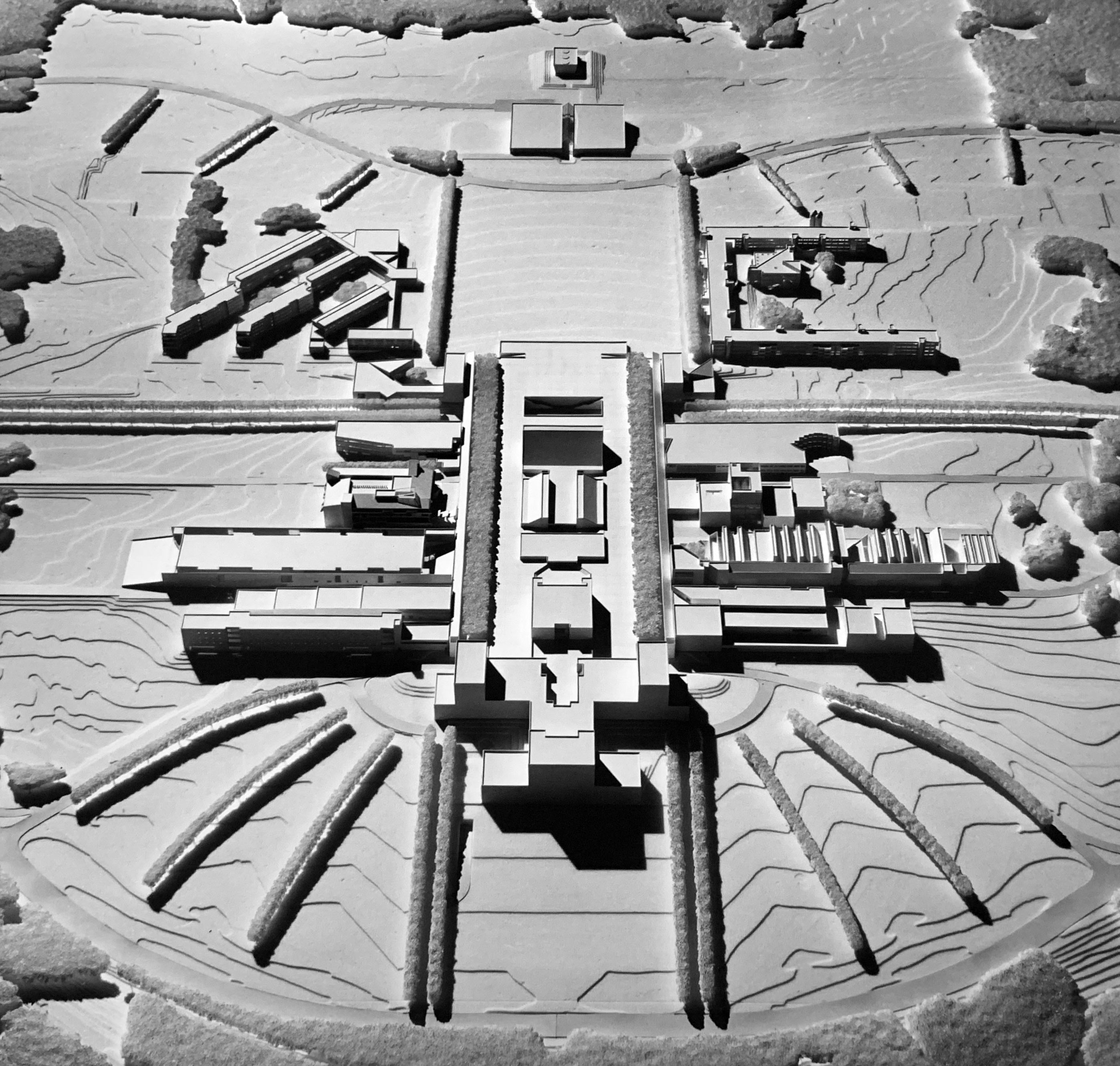The image depicts a black and white aerial view of a structured landscape characterized by its uniform, cubic architecture. At the center of the silver-gray scene stands a prominent rectangular building, surrounded by a network of diagonal lines that hint at the area's planned layout. Flanking this central building are additional structures, each unmarked and blocky in appearance, contributing to the overall industrial aesthetic. The surrounding landscape features orderly rows that may represent hedges and trees, although their square, uniform shapes impart a less organic feel. At the bottom of the image, darker gray vertical arches form a semi-circle, adding a distinct architectural element. The entire scene is devoid of color, relying on varying shades of gray and the play of shadows to create depth and detail. The top of the image showcases two square rooftops, beyond which a denser cluster of tree-like shapes can be seen. Overall, the image presents a stark, monochromatic environment that could suggest a variety of interpretations, from a futuristic cityscape to a meticulously organized complex.